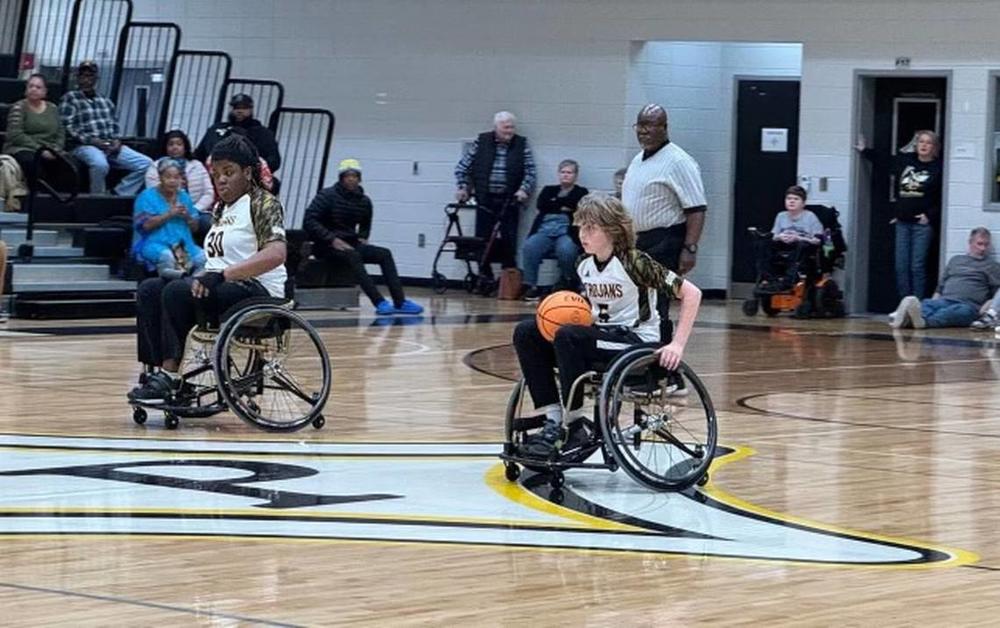In this dynamic photograph capturing the intensity of wheelchair basketball, two young players, likely aged 15 or 16, take center stage. One is dark-skinned and the other light-skinned, emphasizing the diversity within the team. Both athletes are seated in specialized athletic wheelchairs with tilted wheels, designed for agility and speed. The light-skinned player at the forefront has the basketball securely clamped between his knees, poised in mid-drive, seemingly aiming to advance towards the hoop, even though the goals are not visible in this gymnasium's central area. The game scene is vibrant, with blurred motion suggesting a leftward movement.

In the background, a set of populated bleachers underscores the community support for the event, while additional spectators sit on the gymnasium sidelines, creating a lively atmosphere. Among them are another child in a wheelchair, an elderly man with a walker, and a vigilant coach on the gym floor, his eyes trained on the young athletes, ready to offer guidance. The image beautifully encapsulates the spirit of inclusivity and the competitive essence of wheelchair basketball.